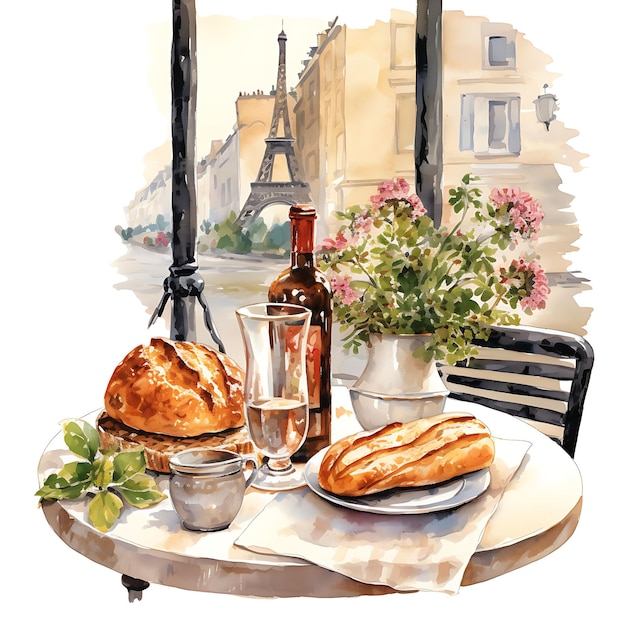The image is a highly detailed watercolor painting of a Parisian scene. At the forefront, there's a small, round beige table with a chair next to it. On the table sits a variety of items: a plate with a round loaf of bread and a half-cut baguette, a glass of water, a cream-colored, grayish small container possibly holding sauce, and a tall, shiny brown bottle of wine. Additionally, there's a white vase holding a bouquet of pink flowers and green leaves. The setting appears to be outdoors. In the background, a row of beige buildings frames the iconic Eiffel Tower, which is visible peeking between the structures. The painting's realistic style beautifully captures the essence of a quaint Parisian setting.